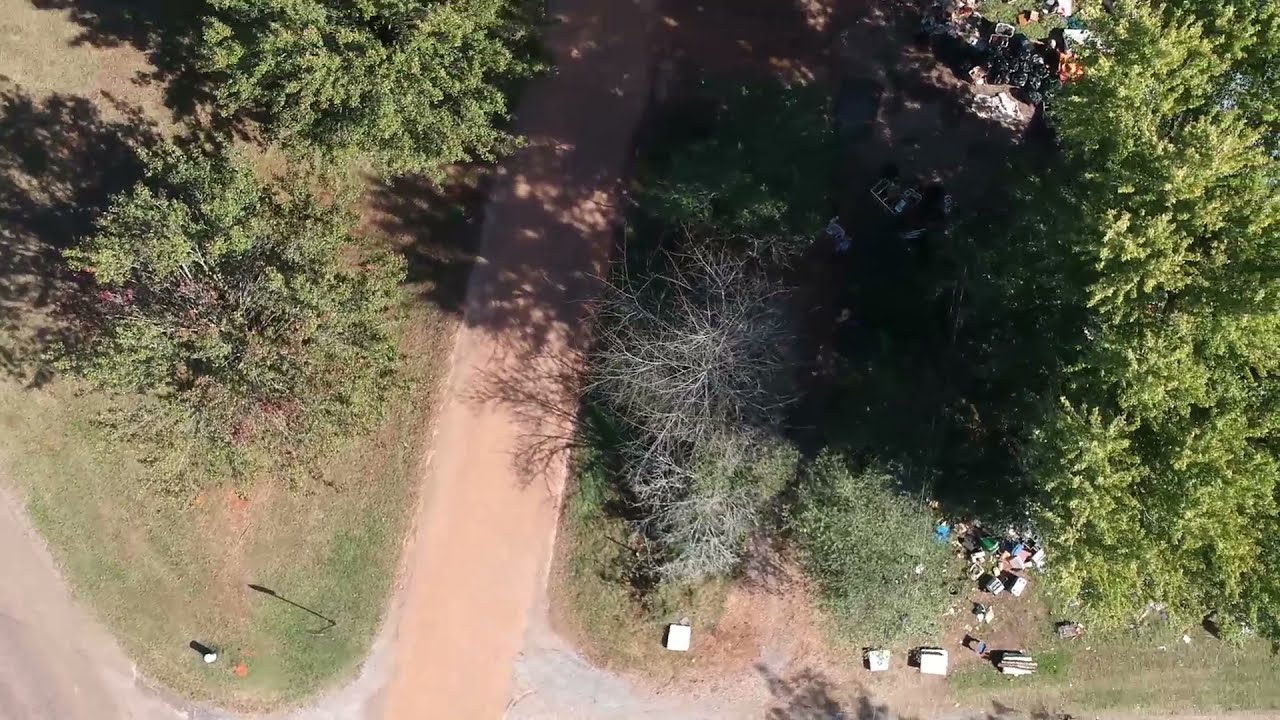This is a color aerial photograph in landscape orientation, depicting a property characterized by intersecting dirt roads and a mix of native grass and exposed dirt, giving it an unmanicured appearance. At the left side of the image, there are two large trees within a triangular island of grass, bordered by a cone-shaped grass area and another dirt road. Centrally, a dirt road runs from the bottom left to the top right, slightly left of center. To the right of this road, the property features multiple trees, some of which are barren and potentially in poor condition. The property itself appears cluttered, with bins, boxes, buckets, and other items scattered in piles, suggesting it might be undergoing construction or has not been maintained for some time. Small white containers are visible near the front of the lot. In the background, a heavy cast shadow extends towards the left side, further accentuating the landscape's realism captured by drone photography.